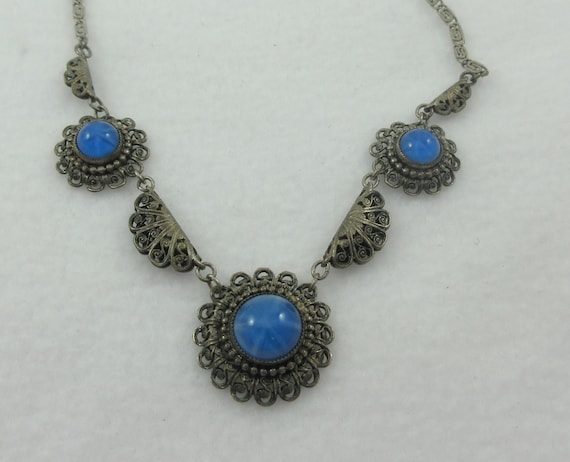This photograph showcases an intricate necklace displayed against a white background. The necklace appears to be made of a tarnished, dark gray metal resembling aged or antique bronze. It features several sapphire-blue jewels, each encased within ornate, swirling metal rings. On the left and right sides of the necklace, two smaller sapphires are set within circular settings adorned with floral and swirl designs. Beneath these, small wing-shaped metal pieces are connected to the sapphires, linking down to a central, larger sapphire encased similarly in an elaborate ring with matching patterned swirls. Above the smaller sapphires, additional wing shapes are attached via tiny chain links. The necklace extends into a substantial and somewhat bulky chain, indicative of an older, more antiquated style. Despite the dull, possibly rusted appearance of the metal, the bright blue of the sapphires lends an elegant and eye-catching touch to the piece.